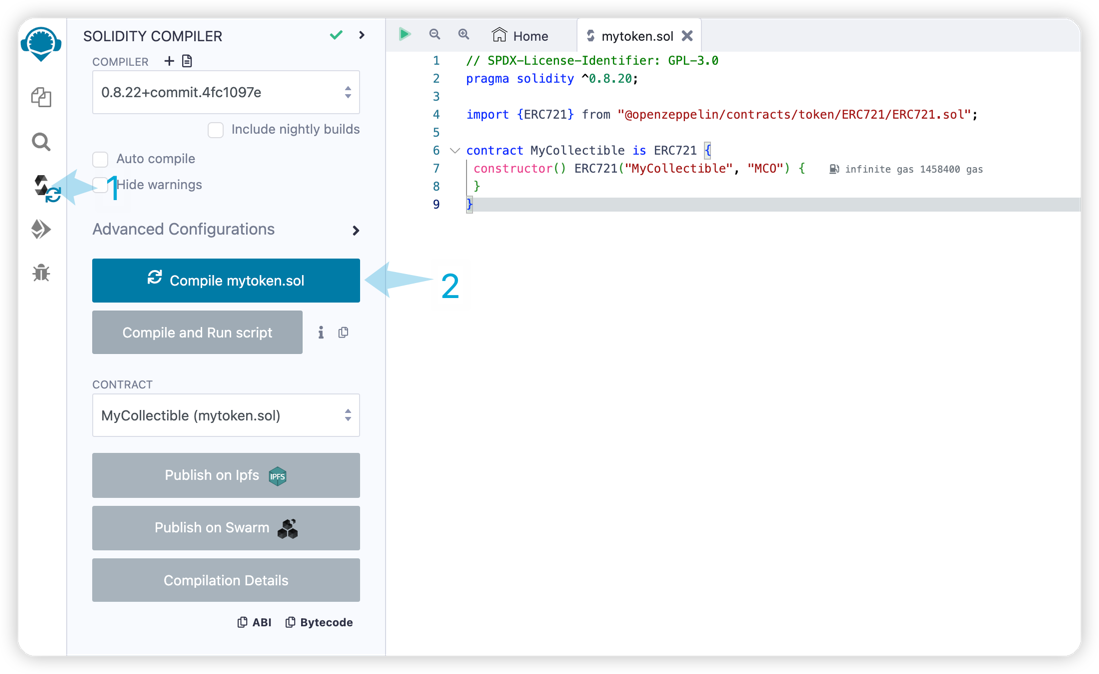The image is a screenshot of a software application with rounded edges and a subtle shadow effect, set against a predominantly white background. The aspect ratio suggests the image is 30-50% wider than it is tall. On the left-hand side, there is a vertical column of six icons. The top icon is a blue, aqua-colored brain wearing headphones. Below this, there is an icon of two folded pages, followed by a magnifying glass. Next is an icon resembling military rank chevrons, with two pairs of arrows pointing to the 11 o'clock and 5 o'clock positions, respectively. Beneath that is a right-arrow icon, and the final icon at the bottom of the column depicts a bug.

To the right of this column is another vertical section with a light blue background. This section appears to be related to a Solidity compiler. Within this area, there is a field displaying a number, followed by the words "commit" and "dot," along with a string of random characters, suggesting it is a place for selecting different options or versions. At the lower right corner of this field is a checkbox option labeled "Include nightly builds."